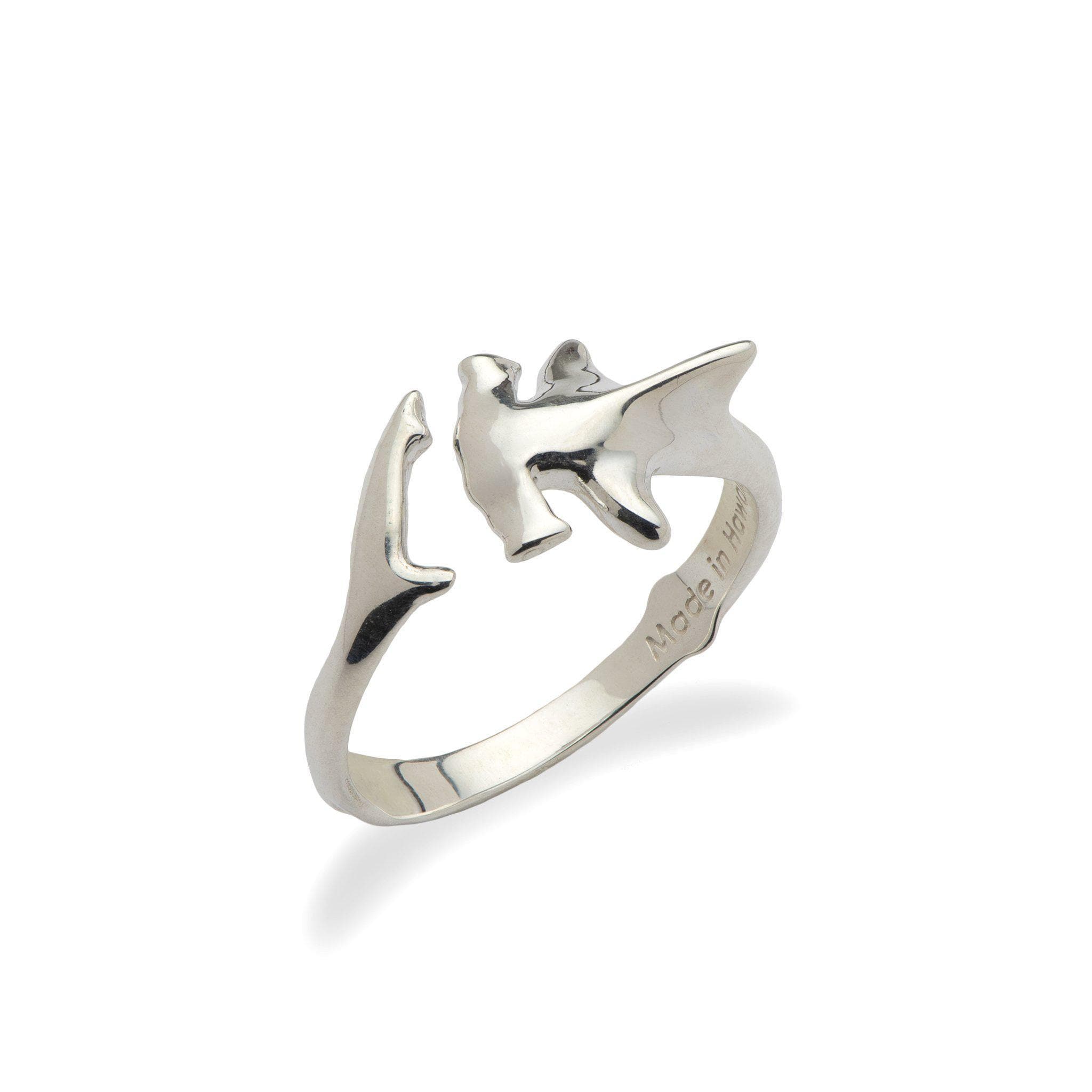The image showcases a striking silver ring designed in the shape of a hammerhead shark. The detailing is intricate: the shark's head, hammerhead fin, tail fin, and body stretch out to form the circular band of the ring, with a noticeable gap between the head and the tail fin at the top. The ring has a glossy, chrome-like appearance, reflecting light brilliantly. On the interior of the ring, an inscription reads "Made in Hawaii," although only the letters "H-A-W-A" are fully visible. The shadow beneath the ring forms a crescent shape on the white background, adding to the visual appeal of the image.